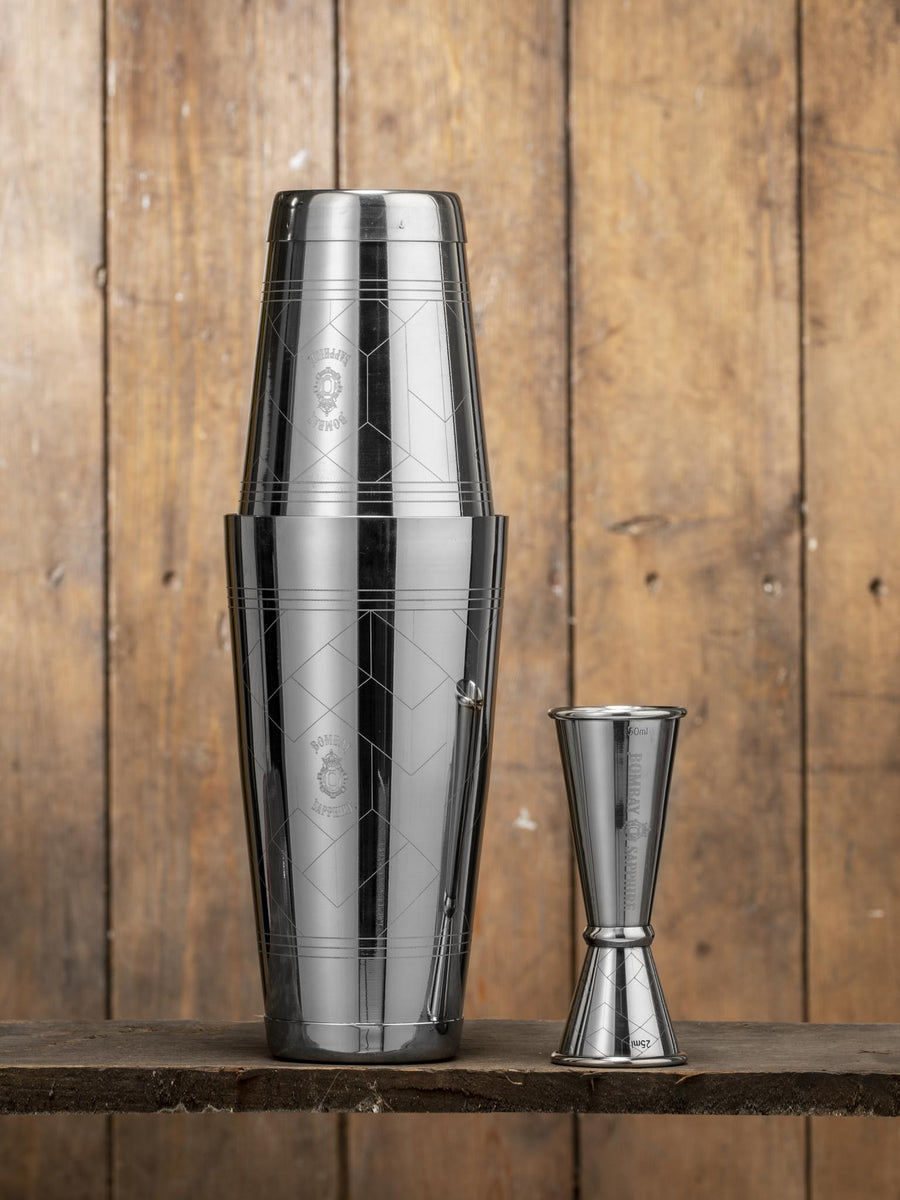The photograph showcases a highly reflective, silver-colored cocktail shaker, adorned with intricate etchings that include patterns of hexagons, squares, triangles, and diamonds. Some markings likely denote a brand, although they are not clearly legible. Positioned to the right of the large shaker is a smaller, similarly reflective metal shot glass, also embellished with etched designs and approximately half the size of the cocktail shaker. Both items rest on a rustic wooden surface, possibly an old wooden table or shelf. The background features a rudimentary wooden paneling, adding to the rustic aesthetic of the scene.